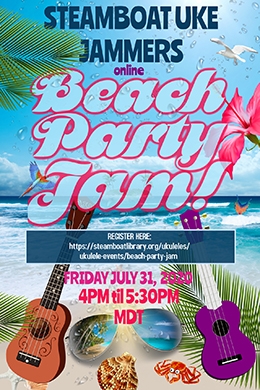The flyer is an advertisement for the "Steamboat Uke Jammers Online Beach Party Jam." The event is scheduled for Friday, July 31st, 2020, from 4 p.m. to 5:30 p.m. MDT. The background features a vivid beach scene with white sand, ocean water, tropical birds flying in the sky, and bubbles scattered throughout. Two guitars, one brown and one purple, appear on the left and right sides respectively. The scene is adorned with a red crab, a brown seashell, a pink tropical flower, and a pair of sunglasses reflecting the ocean and palm trees. The headline "Steamboat Uke Jammers" is displayed at the top in blue text, followed by "Beach Party Jam" with an exclamation mark in red text. Additional details, including the registration link at steamboatlibrary.org/ukuleles/ukulele-events/beach-party-jam, are also provided in the flyer. The entire image has the dimensions of a magazine cover.